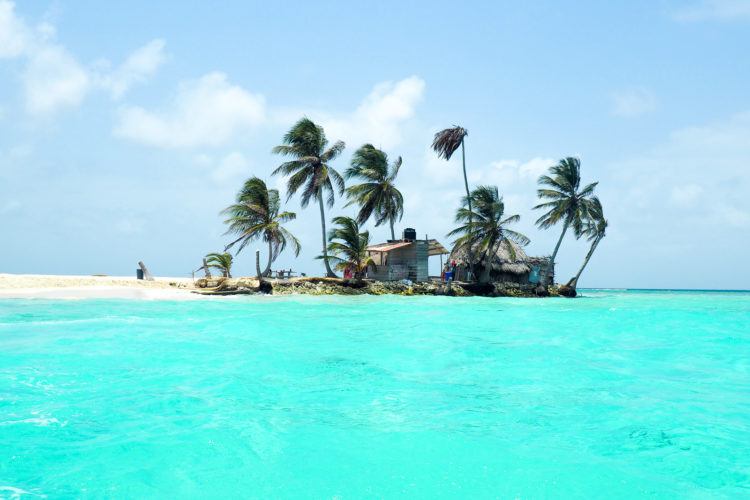In this captivating tropical scene, the foreground is dominated by a bright, almost fluorescent teal water, covering approximately 40% of the image. This clear and inviting aqua blue water transitions into a darker hue further out, emphasizing the depth of the ocean. Just below the center of the image, a sandy peninsula extends horizontally, culminating in a cluster of seven to eight windswept palm trees. These trees partially obscure a humble property consisting of two huts—one appears to be constructed with wood, while the other boasts a roof made of straw or fibrous material, evoking a rustic charm.

Among the palm trees and huts, there seems to be a lone figure standing on the sand, though it might be an object mimicking a human silhouette. The entire setting is bathed under a brilliant blue sky adorned with a few drifting clouds, suggesting a breezy day as indicated by the swaying palm fronds. This serene, isolated beach scene, devoid of any text or animals, whispers of a remote haven, perhaps a hermit's retreat, somewhere in the tropical Keys.